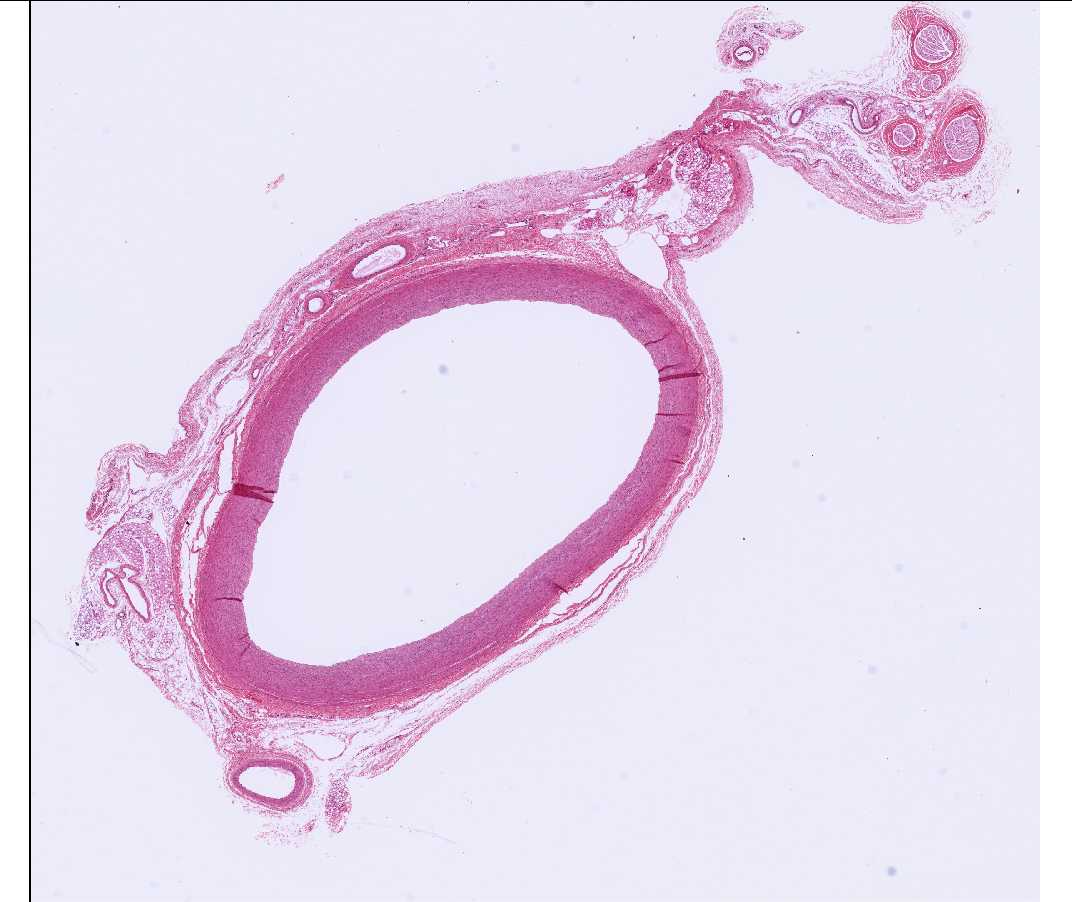The image features a detailed close-up view in a pale white-gray background, resembling a microscopic slide, indicating it may be a scientific specimen. Dominating the scene is a vivid, bright pink oval structure, possibly a tissue or cell, which is prominently bordered by a thick tubing-like rim of a similar pink hue. This large oval shape is connected to a smaller, darker pink circle at its bottom. The whole structure suggests an intricate layering and wrapping of tissues, evoking the appearance of a muscle cell or a similar biological entity with a distinct pink, almost purple coloration. Surrounding this central figure are small flecks or specks dispersed on the white backdrop, adding to the microscopic and scientific aesthetic. Despite the abstract and artistic elements, this detailed image offers a compelling glimpse into cellular or tissue-like formations.